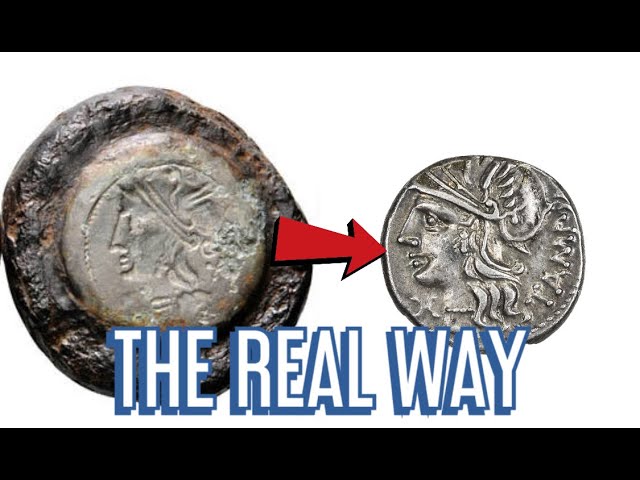The image showcases a digitally captured view of two ancient silver coins, presented against a white background with distinct black horizontal bars at the top and bottom, each about half an inch thick. The entire image is set within a rectangular frame measuring approximately 5 inches in width and 3 inches in height. In the upper and lower sections, the black bands act as borders, while the sides remain open.

In the center of the image, on the left, there is an older, weathered coin that appears to be partially embedded in a dark substance, possibly hardened mud or stone. This coin has a light silver hue and features a faint, raised imprint of a human face, albeit somewhat smushed and indistinct. A red arrow points rightward from this coin to another smaller coin positioned on its right.

The coin on the right is more detailed, depicting a Roman or Grecian figure with a pronounced straight nose and possibly a helmet, highlighting a more refined and clear embossing. Unlike the first coin, this one is free from any surrounding dark material, showcasing a smoother, cleaner finish.

Below this central imagery, just above the bottom black bar, bold white text with a blue-gray shadow effect prominently reads "The Real Way," emphasizing the contrast and evolution between the two coins displayed.